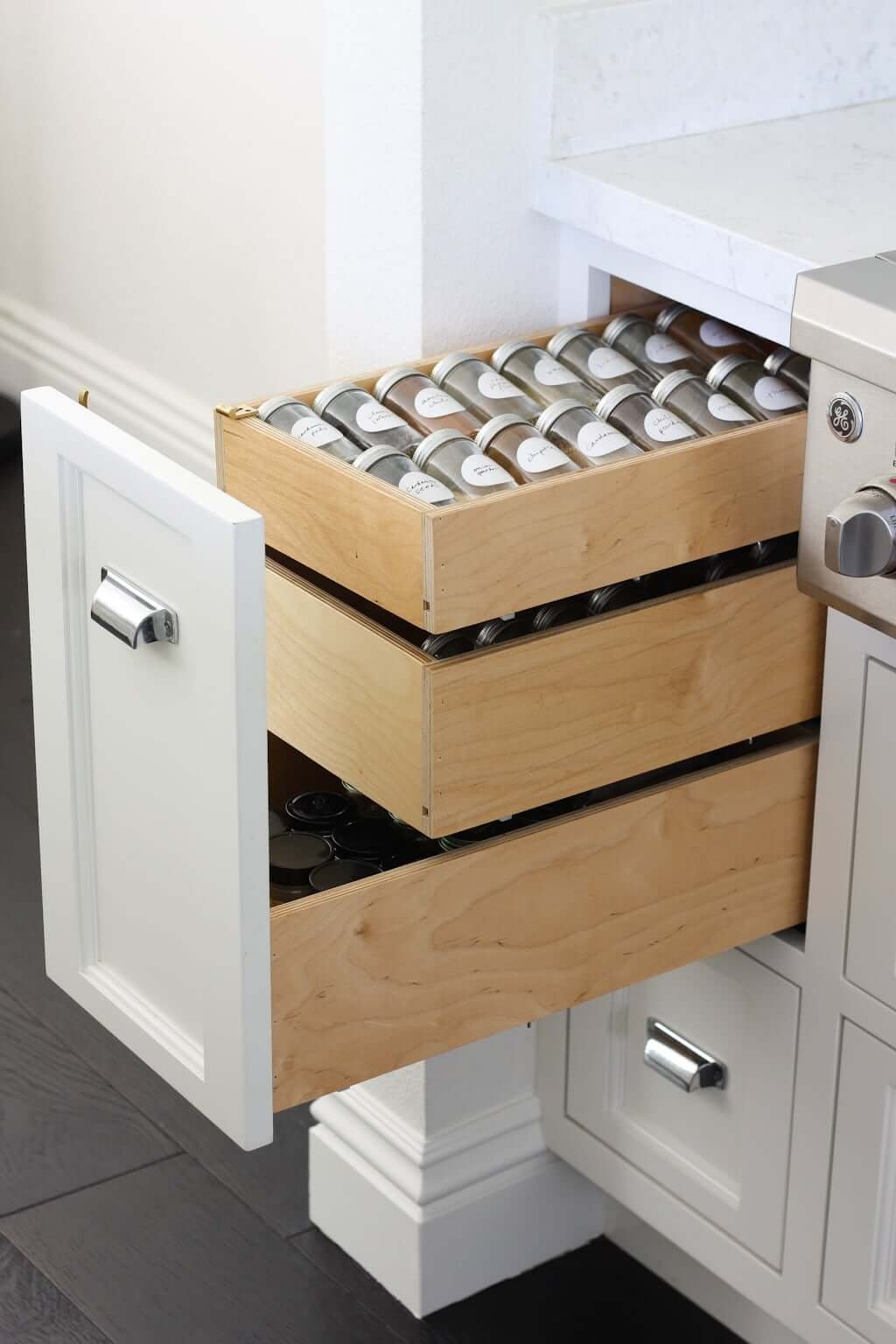The image depicts a small, well-organized kitchen with white walls and cabinetry. Central to the scene is an interesting white cabinet with a large (about four feet high) rectangular drawer and three internal compartments, accessed through a front metal handle. These compartments reveal a neatly arranged collection of spice jars, each with silver caps, suggesting an organized and accessible storage solution. The inside of the drawer features beige wood grain, contrasting the white exterior. Below the large drawer is a smaller, square cabinet resembling the top left of an oven, complete with a knob. The entire setup is designed for convenience, positioned likely near an oven or stove, making it easy to access spices and other kitchen essentials without reaching or searching.